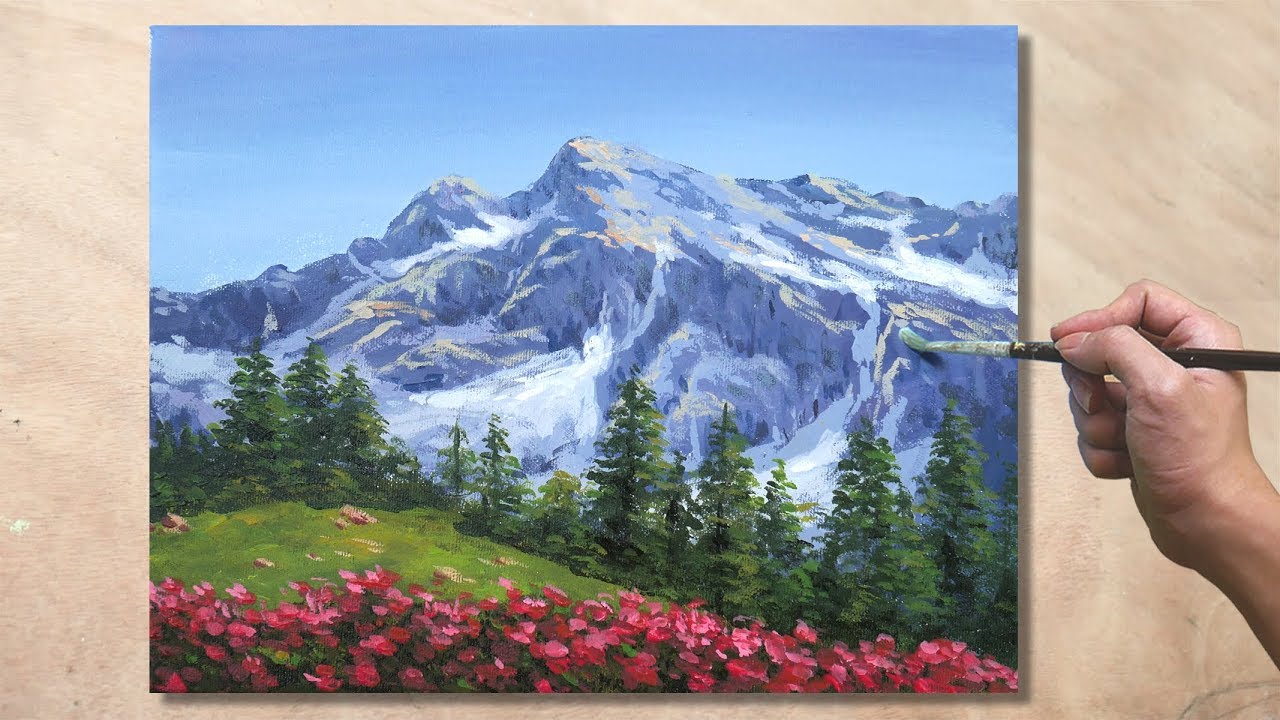In the photograph, a person is seen painting an enchanting landscape. Positioned on a tan, likely wooden surface, the painting captures a mesmerizing scene of towering, snow-covered mountains with bluish-gray hues in the background, highlighted by at least two prominent peaks beneath a clear blue sky. Below the mountains, verdant pine trees spread out, rolling into green grassy fields dotted with rocks. The foreground bursts with the vivid colors of pinkish-red flowers, akin to poppies, stretching across the expanse. The painter’s hand, located on the right side of the image, holds a paintbrush with a dark handle and a chrome ferrule, applying final touches to this impressionistic masterpiece.